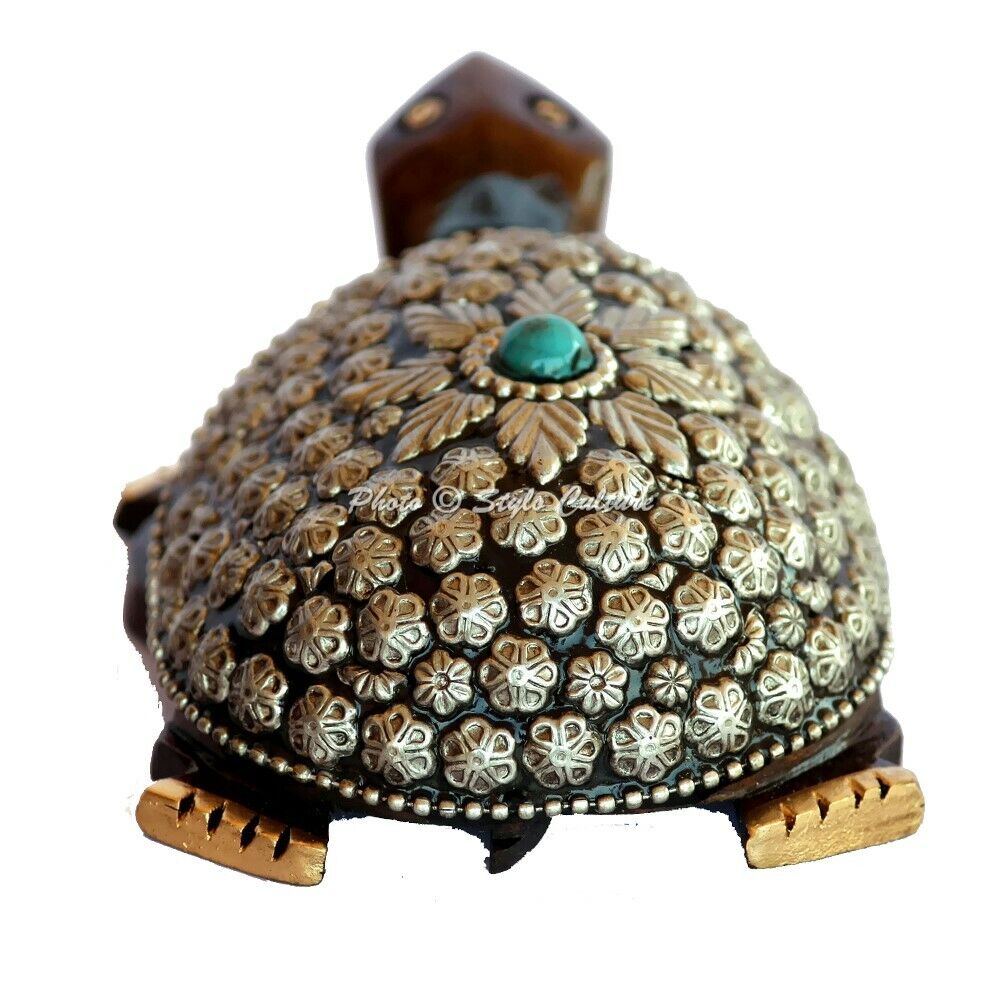The image showcases a detailed and ornate figurine of a turtle primarily made of metal. The turtle's head is turned away from us, displaying a rich wooden color and adorned with gold eyes, although the precise details of the eyes are blurred. The turtle’s feet are gold with intricate indents to indicate toes, and a small black tail is visible from this rear perspective. 

The shell of the turtle is an intricate masterpiece, primarily brown, embellished with closely packed, miniature flower petals that give a blanketing effect. These flowers have a silvery pewter or gold hue. Dominating the top of the shell is a distinct turquoise or teal button encircled by a gold floral pattern and leafy designs that add to the ornamental beauty. The various elements of the shell, ranging from small blossoms to plant leaves and scallops, amplify the figurine’s elaborate craftsmanship and rich textures.